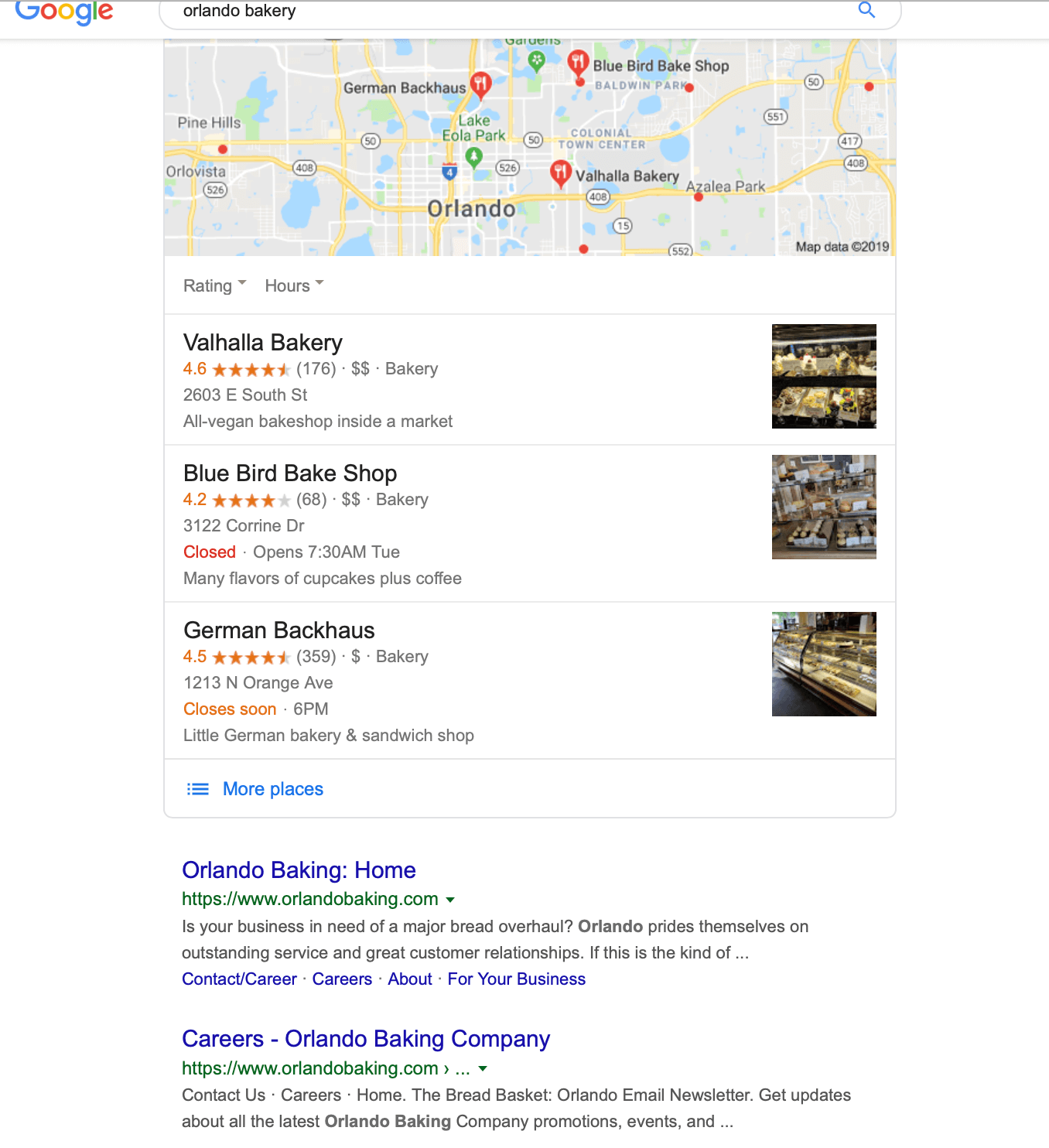The image captures a Google search page. At the top, the vibrant Google logo is displayed in its signature colors: blue, red, yellow, blue, green, and red. Below the logo, the search bar reads "Orlando bakery," accompanied by a blue magnifying glass icon on the right.

Prominently featured is a small rectangular map of the Orlando area showcasing various roads, small lakes, ponds, and the notable I-4 highway. 

The primary search result highlights Valhalla Bakery, located at 2603 East South Street. This all-vegan bake shop is situated inside a market and is marked by a modest price point of $2. The image includes a visual glimpse of some options available in a well-lit display case.

Following Valhalla Bakery, Blue Bird Bake Shop emerges as another option, boasting a 4.2-star rating. However, it is currently closed and set to open at 7:30 AM on Tuesday. This bakery is known for its diverse array of cupcakes and coffee.

The last notable result is German Bockhaus, which holds a strong 4.5-star rating. They are approaching their closing time at 6 PM.